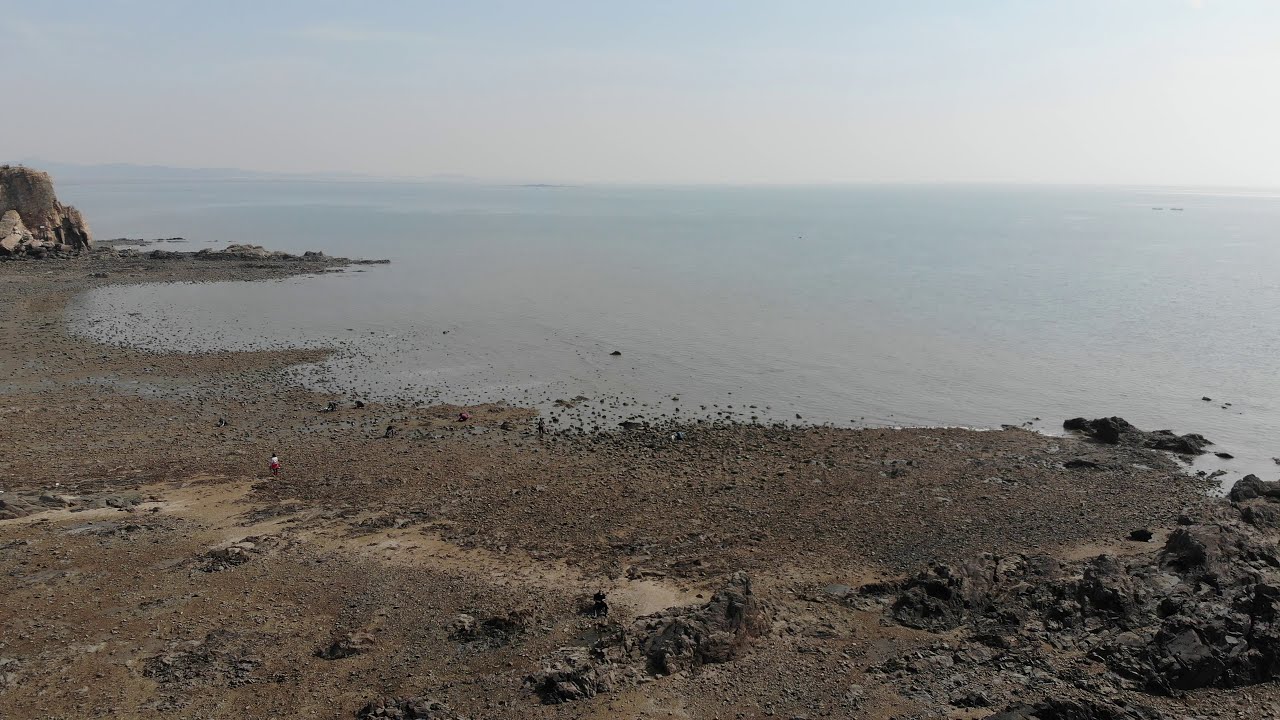In this rectangular horizontal photograph, we see a lakeshore on a dreary, overcast day, with the sky cloaked in gray, casting a wan light over the scene. The water, a mix of blue in the distance and a muddy brown near the shore, stretches out with an endless horizon, fading into the foggy gray sky without a distinct line. The shore is a patchwork of bare dirt, rocks, and gritty mud, suggesting it might flood occasionally, perhaps erasing any hint of vegetation. The scene is muted and fuzzy, lacking sharp sunlight, imbued instead with a foreboding twilight as sunset is close but not quite arrived.

On the far left edge of the image stands a house or similar structure, perched on a small promontory jutting into the water, lending a solitary human touch to this otherwise stark natural landscape. Dominating the rocky, rugged beach in the foreground is a figure, dressed in red pants and a white shirt, their presence adding a splash of color and human interest to the scene. The rocky terrain is littered with sharp, jagged boulders and rocks, interspersed with muddy patches, making it clear this is not a typical sandy beach. The water appears vast and unending, stretching infinitely towards the horizon, reinforcing the sense of isolation and the raw, untouched beauty of this lakeshore.